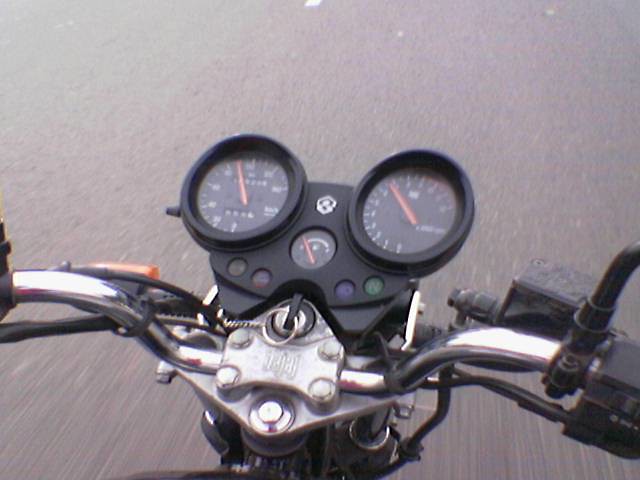The photograph captures a rider's perspective from atop a motorcycle, seemingly on a road trip. The scene is set outdoors on a paved road, with a faint white line in the distance indicating the road's dividing line. From this unique vantage point, the black handlebars of the motorcycle extend into the frame, transitioning into a metallic silver near the center. 

Central to the image is a rectangular silver panel, secured to the bike by four screws— two on each side. Atop this panel, a black key is inserted into the ignition, accompanied by a silver key ring. Directly above this is the motorcycle’s control panel, predominantly black, displaying essential information. 

The speedometer, odometer, and mileage indicator are clearly visible, providing real-time data to the rider. At the bottom of the panel, a smaller, circular gauge indicates the fuel level, showing that the fuel tank is nearly empty. The composition of the photograph, with its attention to detail, immerses the viewer in the experience of riding the motorcycle.